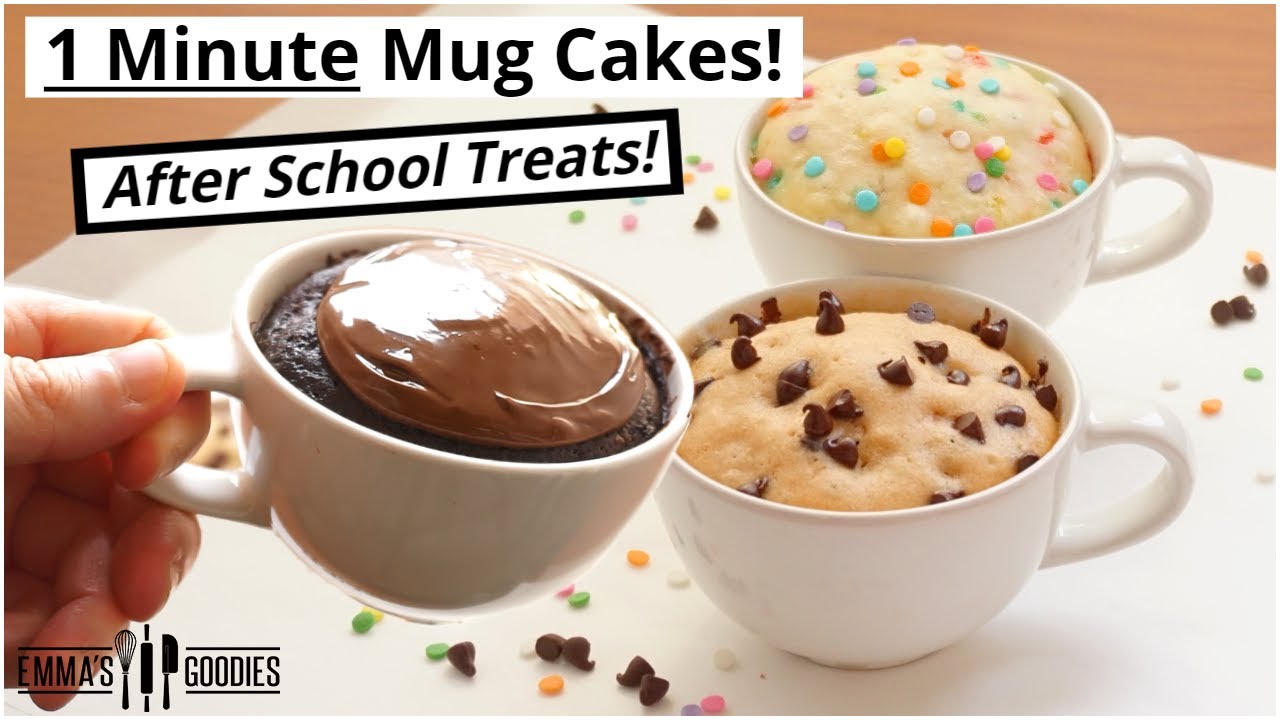The image is a rectangular color photograph with an overlay, resembling something you might find on a food blog or in a recipe section. It features three large white mugs filled with mug cakes, positioned on a white work surface placed on top of a brown table. The text overlay at the top reads "One Minute Mug Cakes, After School Treats" in black and white, while the bottom left corner displays a logo for "Emma's Goodies," featuring a whisk, rolling pin, and spatula.

In the foreground, a hand from the left holds a mug containing a rich chocolate cake topped with chocolate icing. On the table, the middle mug holds a lighter-colored cake embedded with melted chocolate chips. The mug in the background contains a yellow cake adorned with multi-colored confetti candy dots—yellow, white, pink, blue—made of pressed sugar. Scattered around the mugs on the white surface are additional chocolate chips and colorful sprinkles, giving the scene a playful, inviting atmosphere. This image likely serves as a thumbnail for a recipe video, enticing viewers with its vibrant and appealing presentation.